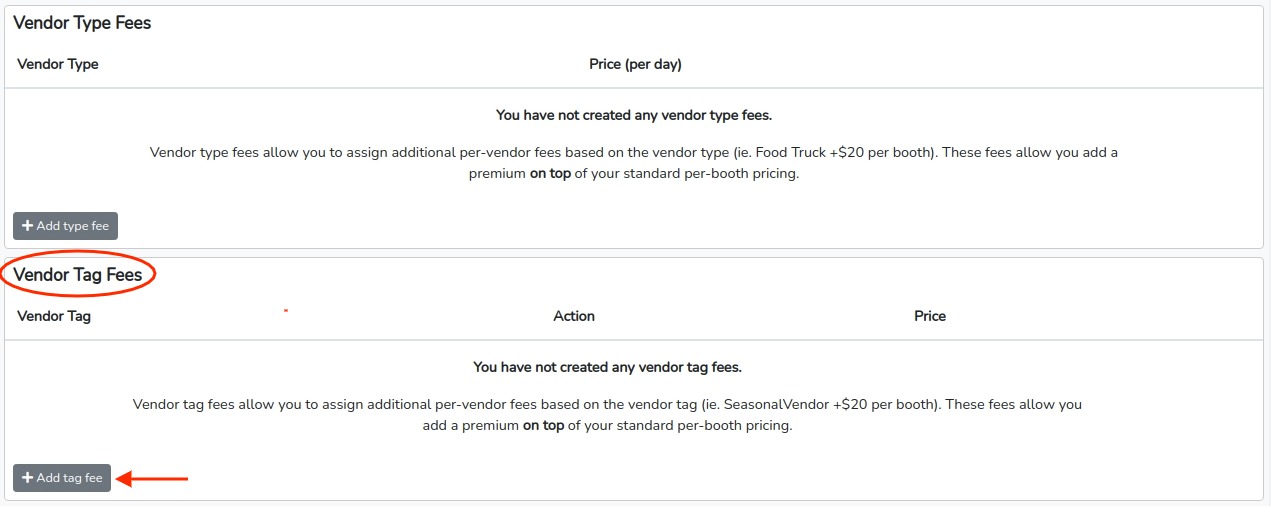This image features a detailed interface from a website, displayed against a completely white backdrop. In the top left-hand corner, "Vendor Type Fees" is prominently written in bold black text. Directly below, in black, is a header that says "Vendor Type" in slightly smaller font.

Moving to the center of the page and slightly to the right, there's a heading "Price (per day)" in black text. A thin gray line separates this section from the next.

Below this divider, a message in black text reads, "You have not created any vendor type fees." Further down, another explanatory text states, "Vendor type fees allow you to assign additional per vendor fees based on the vendor type (e.g., food truck) + $20 per booth. These fees allow you to add a premium on top of your standard per booth pricing."

To the left beneath this text, a gray box is positioned, containing a white plus symbol and the text "Add Type Fee" also in white. Another gray line divides this section from the subsequent part below.

In the new section on the left-hand side, within a sideways white oval shape, it states "Vendor Tag Fees" in black. Directly beneath, "Vendor Tag" is written. To the right of this, and more centered on the page, there is another header labeled "Action," with "Price" to the far right.

Below another gray line, a message appears: "You have not created any vendor tag fees." This is followed by an explanatory note: "Vendor tag fees allow you to assign additional per vendor fees based on the vendor tag (e.g., seasonal vendor) + $20 per booth. These fees allow you to add a premium on top of your standard per booth pricing." Notably, "on top" is in bold.

Under this note, another gray box is present on the left, featuring a plus symbol and "Add Tag Fee" in white text. A red arrow, located on the right side of the gray box, points left towards the text "Add Tag Fee."